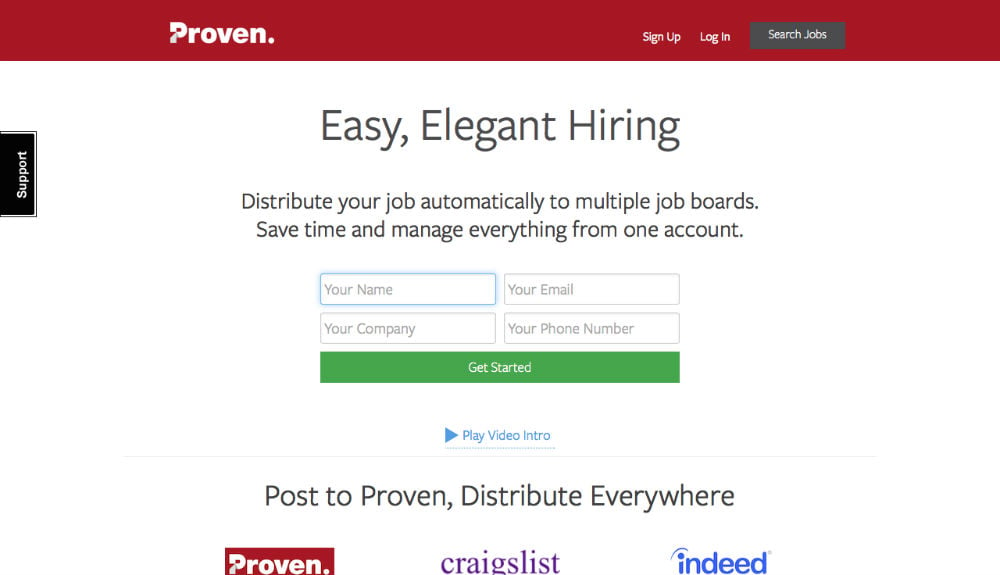This image is a detailed screenshot of the Proven website homepage. At the top left corner, within a red bar, the company's name "Proven" is displayed prominently in white text. On the top right side of the page, there are three buttons: "Sign Up" and "Login," both in white text, and a "Search Jobs" option within a gray box.

In the middle left section of the screen, there is a clickable "Support" button featured in a black box. Centered on the page, the main title "Easy Elegant Hiring" is presented, with a subtitle below it that reads, "Distribute your job automatically to multiple job boards. Save time and manage everything from one account." 

Beneath these titles are four fillable fields labeled for "Your Name," "Your Email," "Your Company," and "Your Phone Number." Below these fields is a green "Get Started" button. Further down, there is a "Play Video Intro" option in blue text, which links to a video presentation.

Further along the page, the text "Post to Proven. Distribute Everywhere" is displayed above logos of three brands: Proven (on the left), Craigslist (at the bottom in purple), and Indeed (on the right in blue). These logos indicate integration or partnership with these brands.

The page appears as an introductory or landing page, characterized by its structured layout and clear call-to-action elements, though all four input fields are currently unfilled.